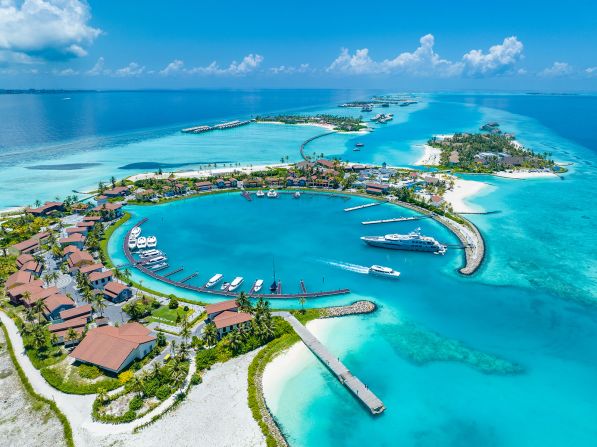This photograph captures an aerial view of a stunning resort set on a circular island surrounded by the vibrant blue waters of the ocean. The image, taken from about 100 to 200 feet in the air, showcases a scenic horseshoe-shaped island densely populated with around 50 to 100 buildings, all characterized by their white walls and clay-colored roofs. Nestled within the island is a central harbor with crystal-clear waters, revealing the sandbars and rocks beneath.

The harbor functions as a marina filled with a variety of boats, including large yachts, small sailboats, and tour boats, all anchored to the docks extending into the vivid blue water. There is a single outlet from this marina that provides access to the vast open ocean. The island is lush with green lawns, trees, and even stretches of white sand. 

The background of the photo is dominated by a serene blue sky, almost indistinguishable from the water save for a colossal white cloud positioned in the top left corner. It's a beautifully bright and sunny day, making the resort appear as the perfect idyllic getaway.